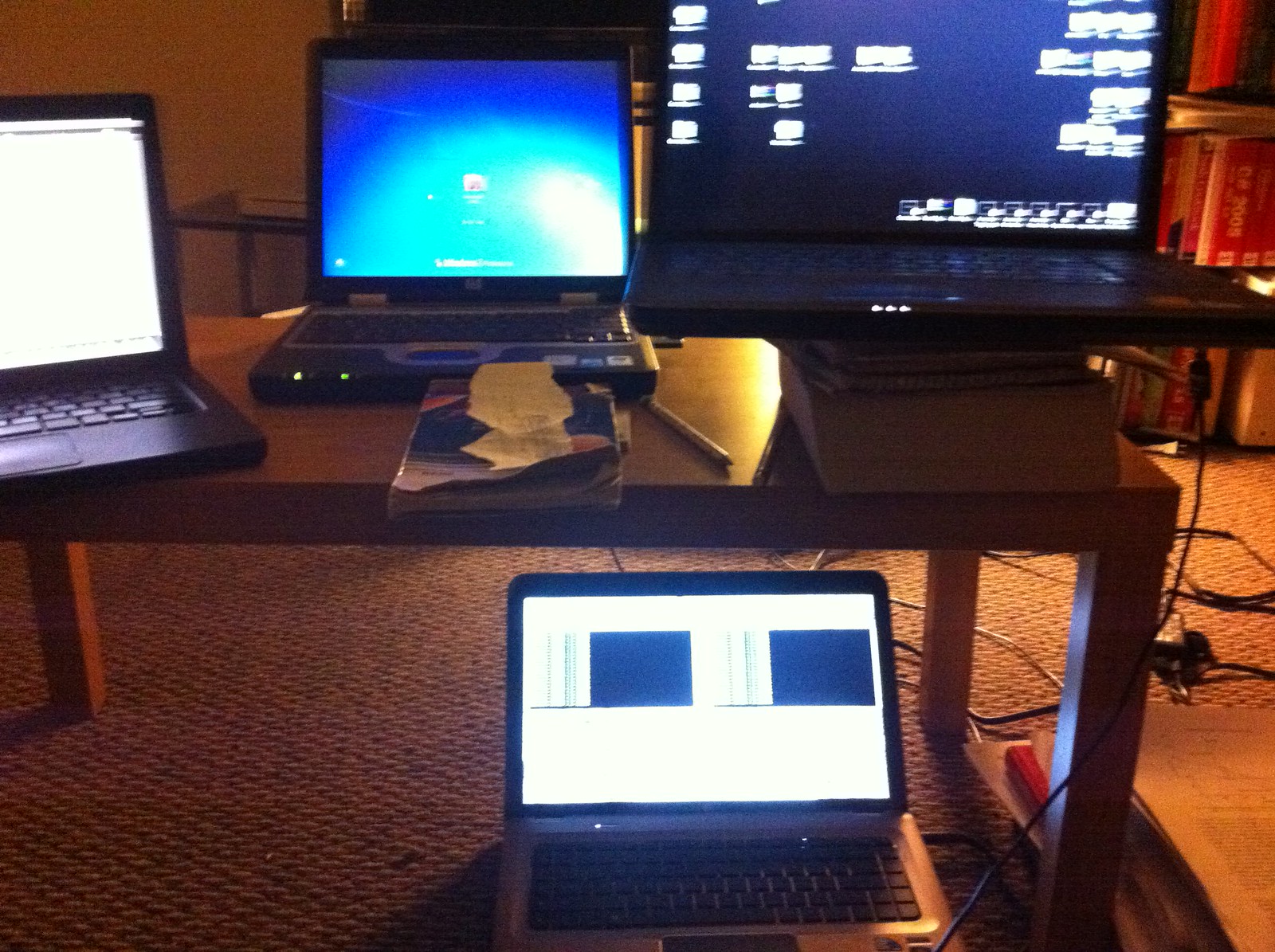The image depicts a cluttered office space centered around a large, light brown wooden coffee table, which is rectangular in shape and stands low to the ground. This table is the primary surface holding an array of technological devices and office supplies. 

Prominently on top of the table are three laptops: a silver laptop resting on a stack of books shows a dark blue screen filled with blurred icons; a smaller black laptop displays a Windows login screen over a blue background, complete with green indicator lights and labels for the processor and operating system; and another black laptop on the right side is turned on with an unidentified black webpage or screen.

Below the coffee table, placed on the brown carpet that is adorned with diagonal patterns and divots, there is an additional silver laptop. This laptop displays an open Excel sheet on its left side and a blank black space on its right. The scene is completed with numerous black, gray, and white cords scattered primarily on the right side of the coffee table.

In the background, there is a bookcase filled with various books, many of which have red bindings, and a Nintendo Wii console partially visible with its white body and black faceplate, adding to the impression of a busy, multi-functional area.